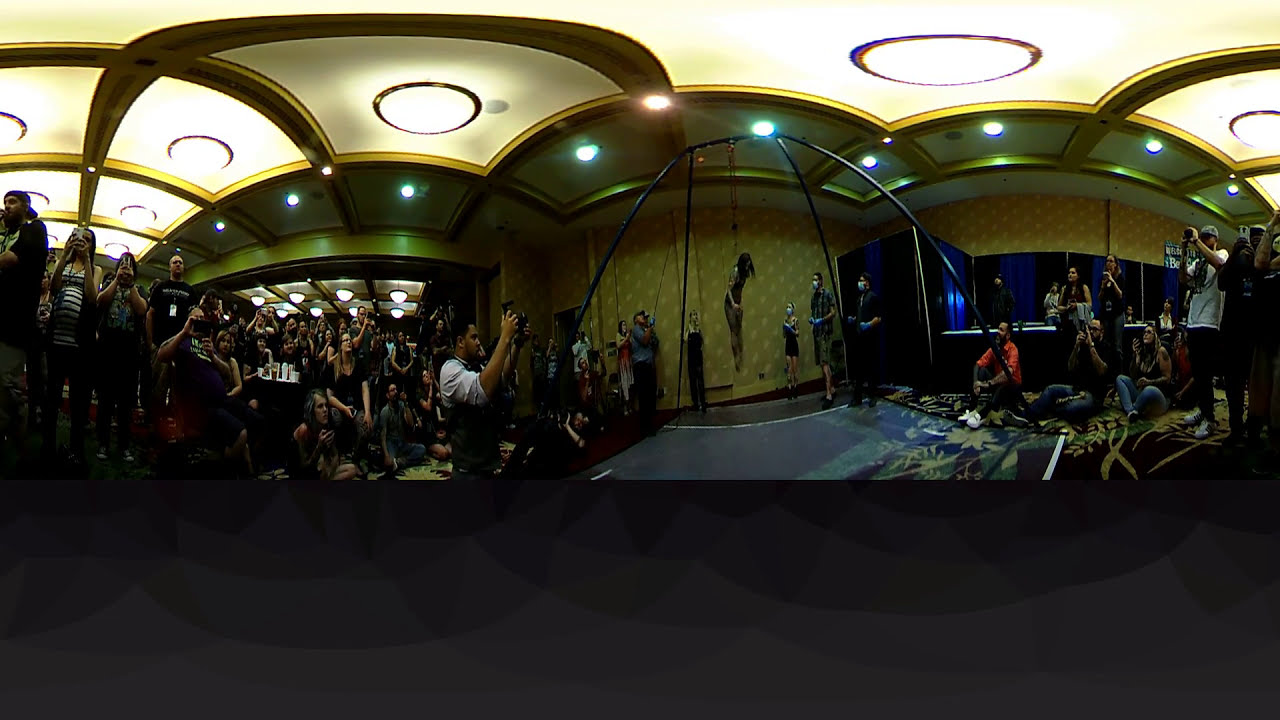Inside a spacious room adorned with a white ceiling featuring decorative gold circles and curved gold metal strips, a large crowd is gathered, giving the sense of an exhibit or event. The walls are a patterned gold, interspersed with white dots, and the floor is decorated with a brightly colored gold, blue, and green carpet. Bright spotlights shine from the ceiling, illuminating the scene. 

In the center of the room, a striking metal apparatus composed of multiple poles arranged in a formation stands out. Suspended from this structure by a rope is a woman with long dark hair, dressed in black stockings and a tight small top, seemingly tied by her back. She hangs above the crowd, who are fixated on her with cameras in hand, capturing the moment. Some attendees are wearing masks and blue gloves, further emphasizing the unusual nature of the spectacle. 

The left side of the image reveals a dense gathering of people, both standing and sitting, particularly in the front where the most eager photographers are positioned. The right side shows a slightly sparser crowd, with some individuals standing around blue tables and backings. The entire scene is bathed in a mix of anticipation and curiosity as if this could be either an avant-garde art performance or something more ambiguous.